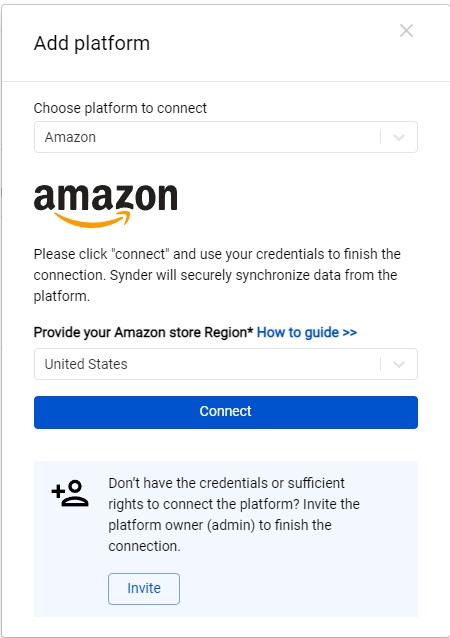The image displays a clean and minimalist screenshot set against a solid white background, bordered by a thin gray line on the top, bottom, and left sides. In the upper left corner, the text "Add Platform" is written in black, while the upper right corner features a light gray "X". Below a thin gray horizontal divider, the text "Choose platform to connect" appears. Directly beneath this is a dropdown menu displaying the word "Amazon". 

Prominently displayed below the dropdown is the Amazon icon, which includes the traditional yellow arrow pointing up and to the right, accompanied by bold black text. Under this, the instructions read: "Please click Connect and use your credentials to finish this connection. Sinder will securely synchronize data from the platform." 

Following these instructions, there is another prompt: "Provide your Amazon store region." Directly below this prompt is a blue hyperlink labeled "How-to guide". Completing the form is another dropdown menu with "United States" as its default selection. The overall layout is clear and organized, guiding the user through the connection process step-by-step.